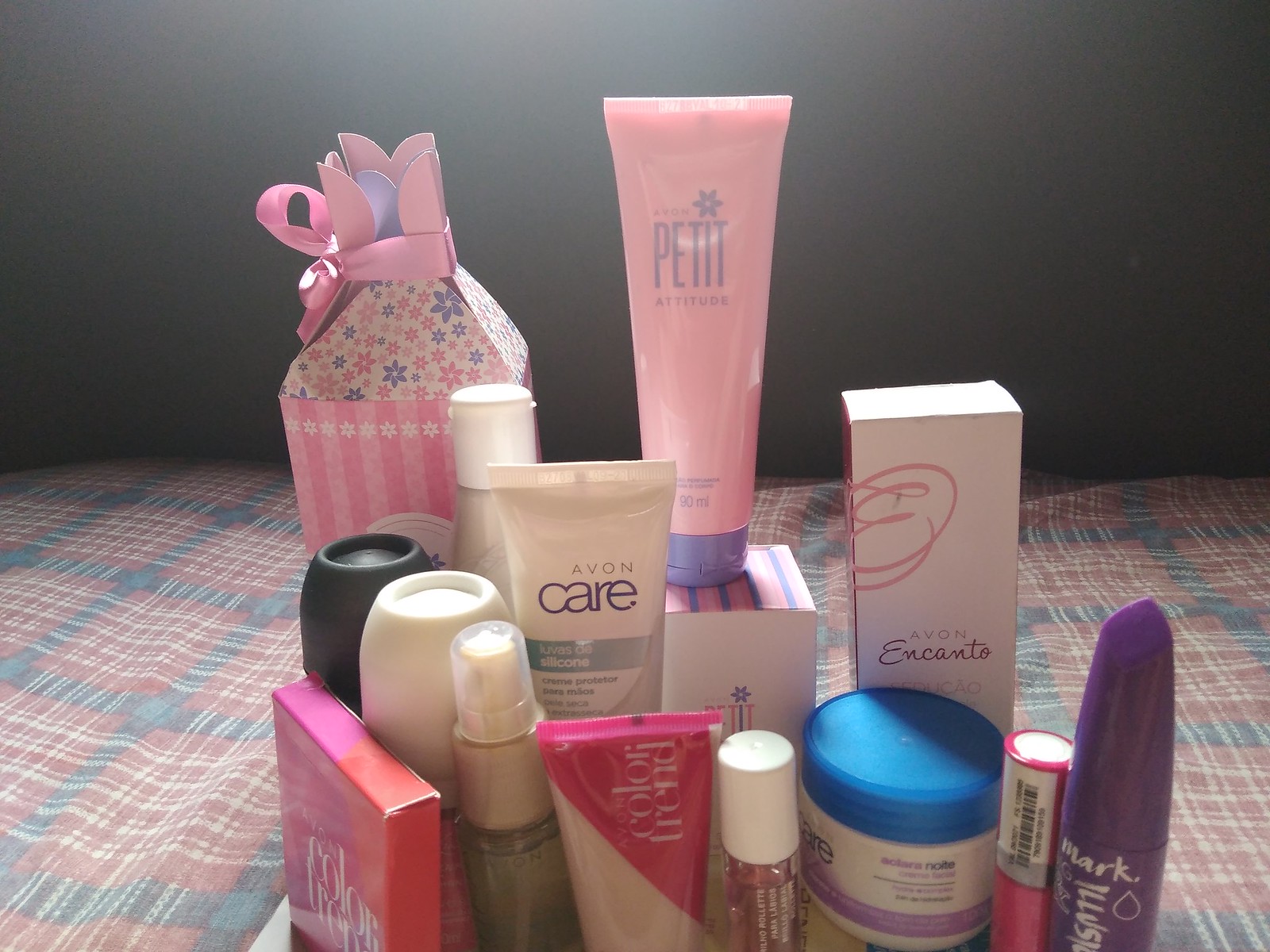In this detailed photograph of skincare products, likely for women, the items are arranged on a checkered sheet that serves as a surface. The sheet features bold grey lines intersected with red blocks and white overlay lines. The background is a muted brown, potentially a wall, headboard, or the backside of a couch. 

The skincare products are clustered together towards the bottom middle of the image. On the bottom right, there is a purple container, possibly mascara, with the readable text "Mark." To its left is a pink tube, which could potentially be a lipstick. Moving further left, there's a cream in a white container topped with a blue lid, its brand unidentified. Behind this cream, a white box labeled "Avon Encanto" is visible.

At the front, there's a transparent glass tube with a white lid, contents unknown. Another plastic tube, marked with a pink triangle on one end and the words "Color Trend," is to its left. Also included is a plastic, see-through spray bottle with a white lid. A small, pinkish-orange box labeled "Color Trend" is positioned next to it.

Additionally, there are two items that appear to be roll-ons, distinguished only by their lids—one white and one black. An "Avon Care" tube is also present, along with a "Petite Attitude" pink tube with a purple lid visible towards the back. Lastly, there is a small, decorated box with flower designs, though its contents are unspecified.